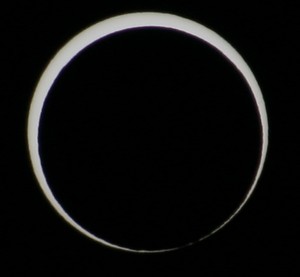The image features a black background with a central graphic that resembles an eclipse. Dominating the scene is a silvery-blue circle that has a subtle bluish tint. Superimposed onto this larger circle is a smaller, solid black circle positioned slightly off-center. The black circle encroaches upon the silvery-blue one, nearly touching its lower right edge and creating a varying band of light; this band of silvery-blue light is narrower at the lower right and much wider at the upper left. The overall effect is that of a visually striking, albeit imperfect, eclipse set against a stark black field.